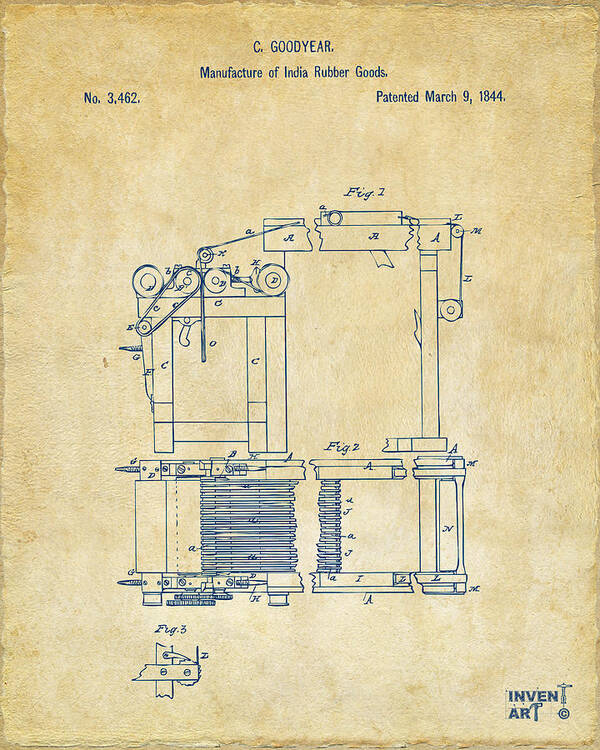This is a detailed engineering drawing of a mechanical device used for manufacturing, created by C. Goodyear, manufacturer of India rubber goods. The drawing is on weathered, brownish paper, originally white, dating back to March 9, 1844, with patent number 3,462. The top of the page prominently features this information in dark blue text. The diagram, also in blue ink, presents two figures labeled 'Figure 2' that detail different aspects and operations of the device. It incorporates various components like pulleys, belts, flywheels, rods, and screw-like structures, indicative of its rotational and mechanical functions on a factory floor. Rubber blanks enter from the bottom of the device, suggesting part of the rubber manufacturing process. Notably, an area within the illustration resembles an electrical coil positioned between two rods. The lower right-hand corner of the drawing is marked with the phrase "Invent Art," adding a decorative touch to this historical patent document.